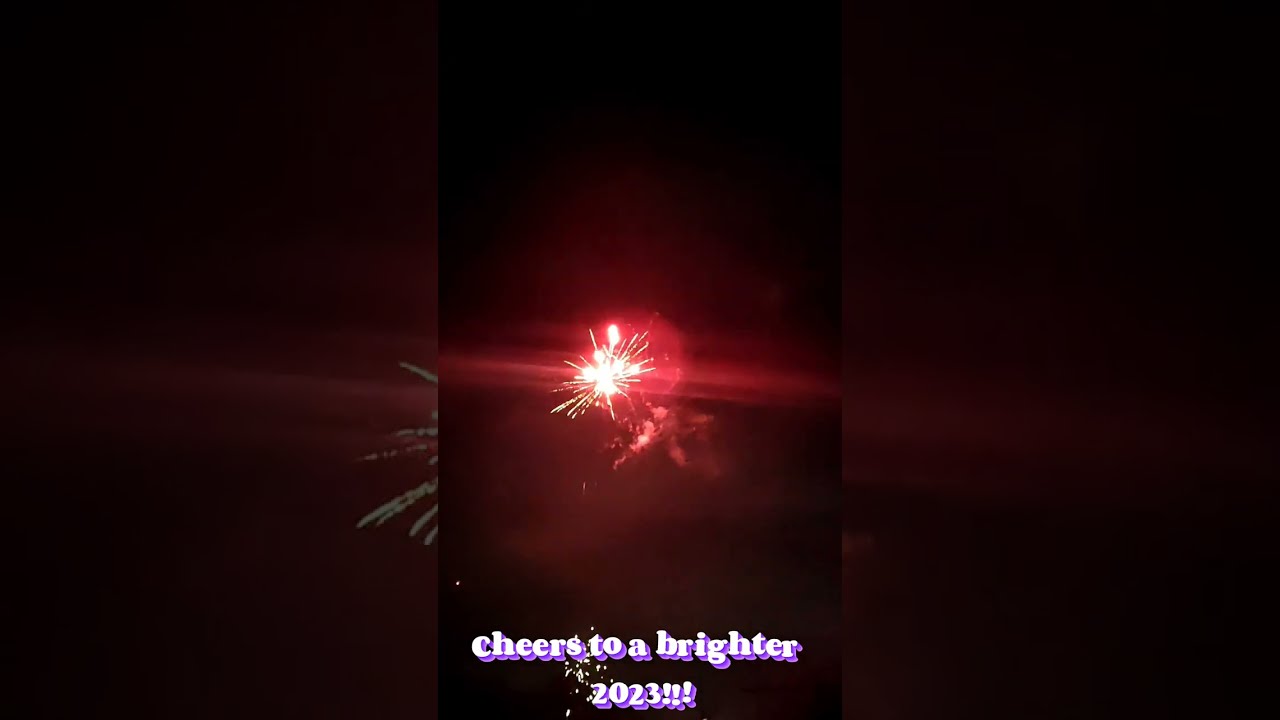The image showcases a dramatic night sky dominated by a bursting firework. The background is predominantly black, accentuating the vivid display at the center. This central firework explosion is primarily white, spewing streaks of light in all directions and accompanied by a glowing red flare that illuminates a surrounding smoke cloud, casting a red hue across the scene. Behind this firework, there is a faint outline of a tall, rectangular black building. The overall scene is mirrored vertically in larger rectangular boxes on either side of the central image, but these side images are zoomed in and darker in shade, creating a layered effect. At the bottom center of the image, two lines of bold white text with a subtle dark purple drop shadow read: "Cheers to a brighter 2023!!!"